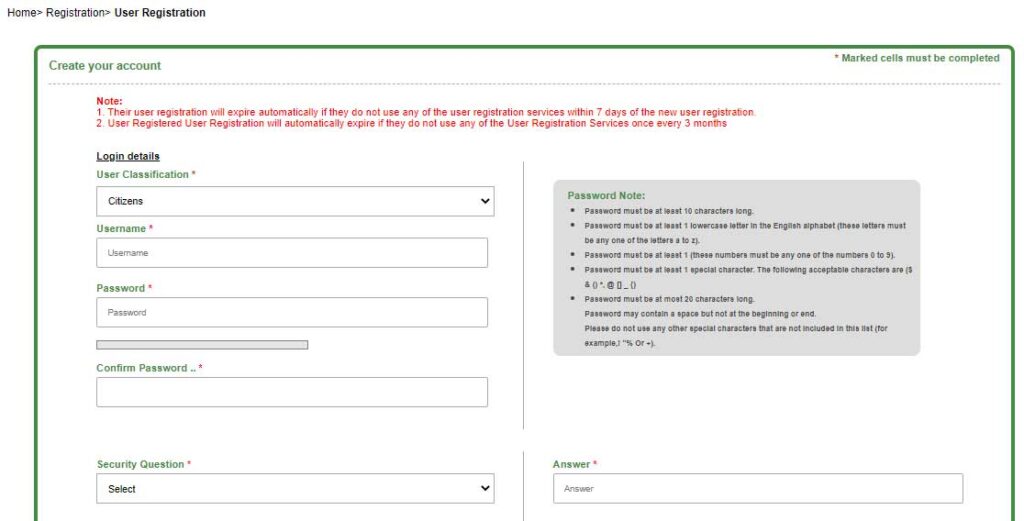The image depicts a partially visible webpage, primarily showcasing a user registration form. On the top left corner, there is a breadcrumb navigation trail that begins with "Home," followed by an arrow pointing to "Registration," and another arrow leading to "User Registration." Below this navigation trail, the header "Create Your Account" is prominently displayed, bordered by a green line that runs vertically and horizontally around the section until the point where the image is cut off.

To the right of this header, the text "Marked cells must be completed." is visible, separated from the rest of the section by a dotted line. Below this, there is text in red font starting with "Note:" followed by two numbered points, each containing a sentence of information.

Further down, there is a section labeled "Log and Details," which is underlined in black font. Underneath this section, entitled "User Classification," there is a star symbol indicating important information. The form includes fields such as "Citizens" with a drop-down arrow, "Username," "Password," and "Confirm Password." 

Additionally, there is a rectangular, empty space followed by a "Secret Question" drop-down menu labeled "Select." Adjacent to this, there is a box labeled "Password Note" containing bulleted information relevant to password creation. At the bottom of the form, there is an "Answer" box for entering the response to the selected secret question.

Overall, this detailed registration form is partially captured, revealing an organized layout with specific instructions and fields required for user account creation.